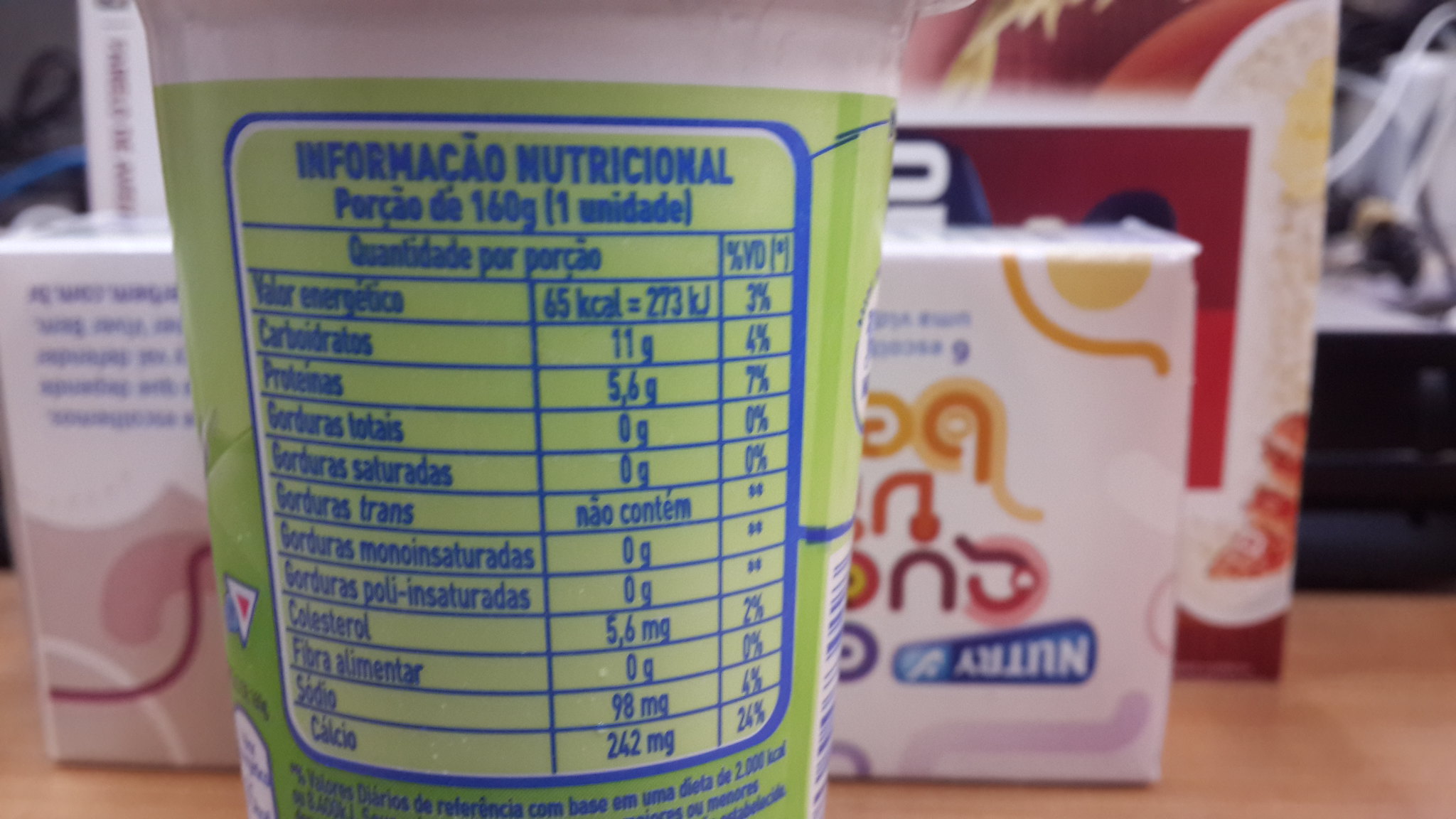This image showcases a lime-green nutritional facts label affixed to a small, round, plastic container resembling a yogurt tub. The label, adorned with light blue trim, lists nutritional information in an unfamiliar language, featuring terms such as "informacado," "nutricicano," and "nutricigan." Positioned next to the container is an upside-down box displaying the word "Nutri." Additionally, part of another box, possibly for Quaker oats or grits, is visible in the background.